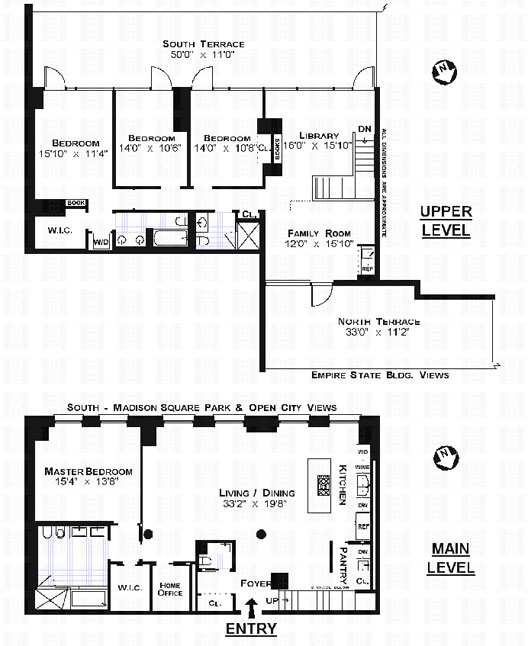The blueprint consists of two detailed floor plans sketched on white paper, both featuring a north indicator pointing to the bottom right corner. The top blueprint is labeled "Upper Level" and depicts three bedrooms positioned either to the top right or top left. Adjacent to these bedrooms on the right is a library. Each room features detailed measurements. At the uppermost part of this blueprint is a designated "South Terrace," measuring 50 by 110 feet. Below the bedroom area, there are multiple bathrooms and a closet. Additionally, there is a family room located to the right of these bathrooms and closet, measuring 12 by 16 feet, with a "North Terrace" adjacent to it, measuring 33 by 11.2 feet.

The bottom blueprint illustrates the main living and dining areas. This level includes another master bedroom and an adjacent bathroom, situated in the bottom left corner. Next to the bathroom is a small water closet, and to its right is a compact home office. The kitchen is located along the right wall, adjacent to the living and dining space. Each room is annotated with precise measurements, delivering a comprehensive overview of the house's layout.